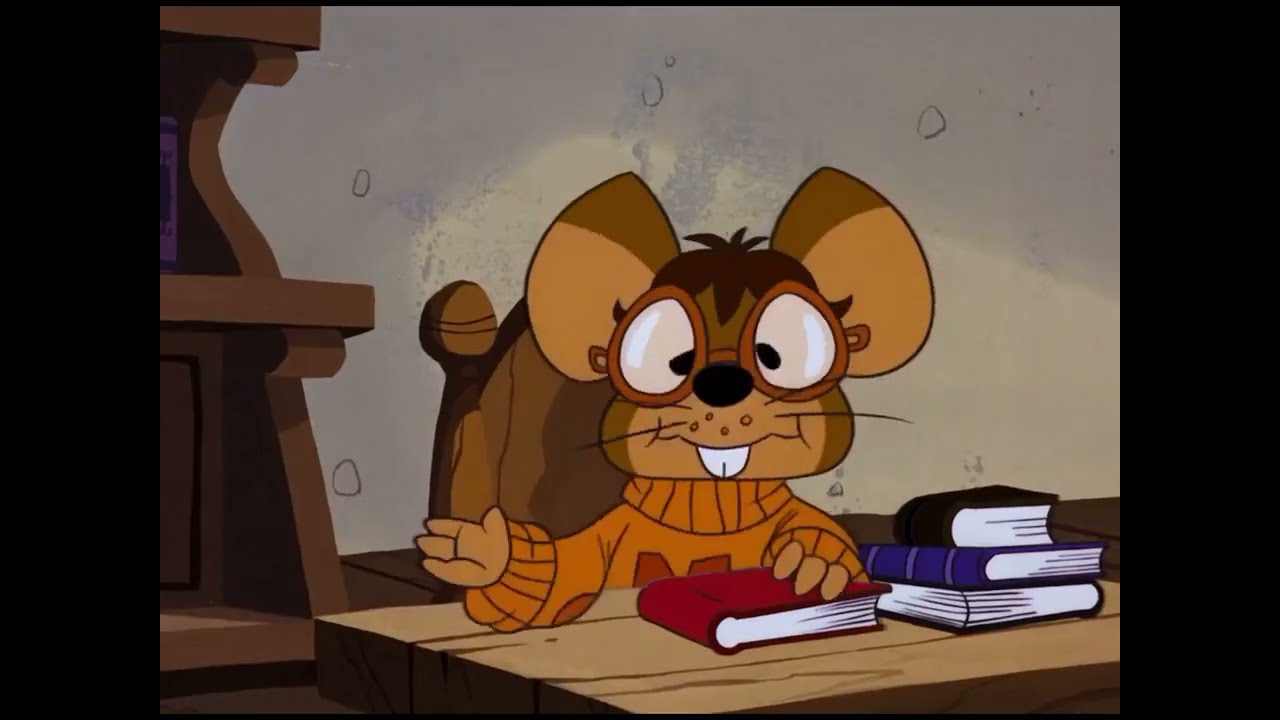The image is a horizontal rectangular frame bordered by vertical black strips on the left and right edges. At the center is a cartoon scene featuring an intelligent-looking mouse with large, light brown ears tipped in dark brown, and wearing orange-rimmed glasses. The mouse has a dark brown face except for the area around the mouth, which is light brown, highlighting two prominent buck teeth. The mouse is smiling slightly and has visible whiskers. It is dressed in a long-sleeve orange sweater with indistinct details on the front and is seated at a desk. The desk is light brown wood and features a stack of three books to the right: a black book on the bottom, topped by a purple book, and then another black book. The mouse's left hand rests on a maroon or red book in front of it while the right hand is outstretched, palm facing forward. The background consists of a grayish wall and a wooden bookshelf to the left, with a purple book partially visible on the top shelf and an empty bottom shelf. Wooden flooring can be observed underneath the mouse and the desk.